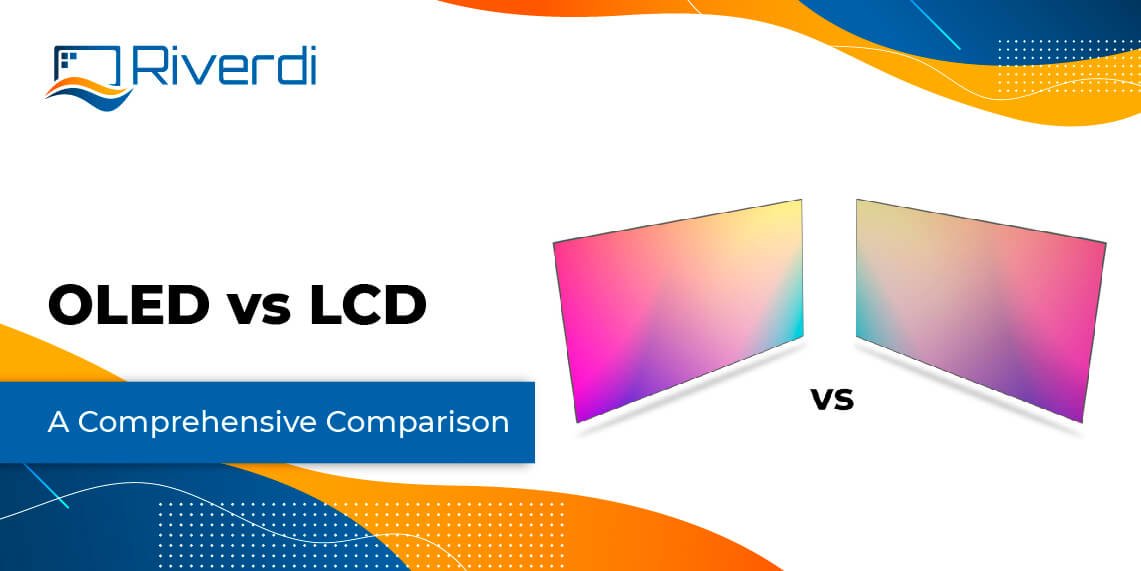The image appears to be an advertisement for a brand named "Riverdy," showcasing a comprehensive comparison between OLED and LCD TV screens. The backdrop is predominantly white, with a curved orange and blue design sequence at the top corner and a series of white dots arranged in an 8-row by 20-column grid. Below this design element is the brand name "Riverdy" in blue technical letters, accompanied by a logo featuring three small squares. The main text includes "OLED vs LCD" in black font and "A Comprehensive Comparison" in white text within a blue box. In the center, two TV screens displaying purple, white, and green colors are positioned to face each other, with the word "versus" between them. Additionally, an orange and blue wave design appears in the bottom left corner, reflecting the style seen at the top. The overall image is colorful, incorporating shades of red, orange, blue, pink, purple, yellow, and teal, creating a vibrant and technical aesthetic.